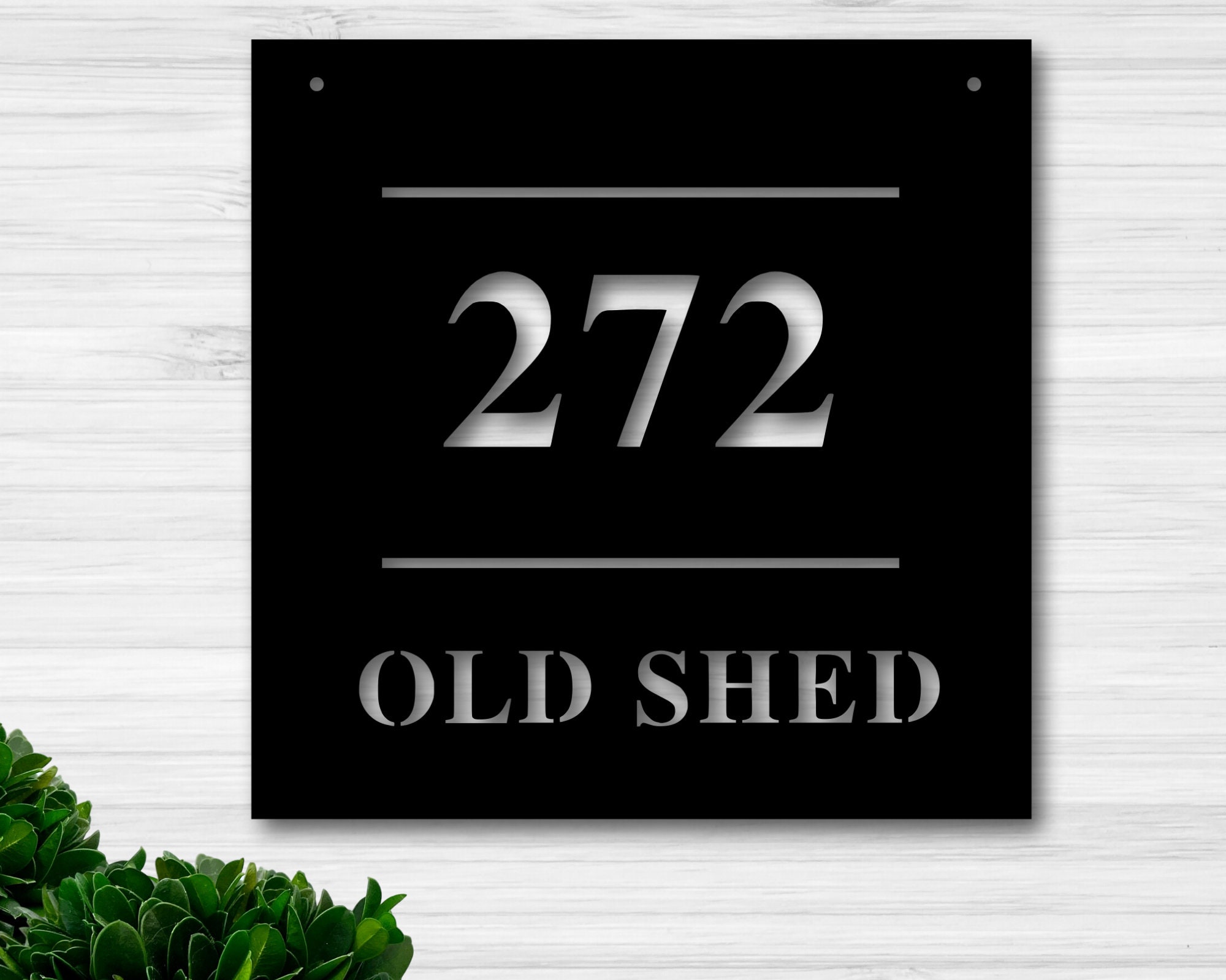The image showcases a black metal sign affixed to the white brick exterior of a house, which has a texture that might also be wood painted white. The sign is bolted to the wall with small gray bolts at each corner and features cut-out characters that reveal the white wall behind it. Centered in the sign, the numbers "272" are displayed prominently, sandwiched between two horizontal gray lines. Below the second line, the cut-out letters spell out "Old Shed." Along the bottom left edge of the wall, a few green bushes with thick leaves grow from the ground, adding a touch of greenery to the scene.